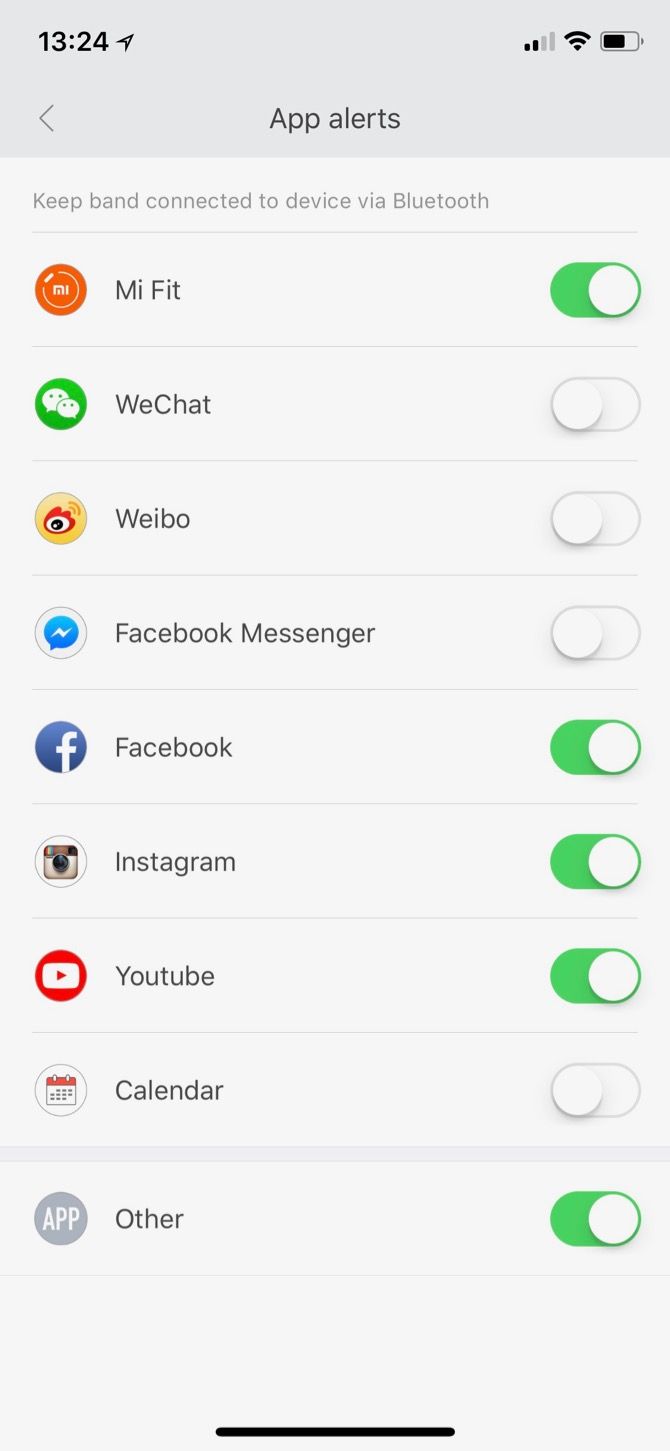The top section of the image has a gray background featuring the text "13:24" in black, with an arrowhead-like symbol pointing diagonally towards the right. Below this, the surface displays two black bars, two gray bars, a white bar, and another black bar. The battery indicator is more than 70% filled, shown in black.

On the next row, towards the left side, there is a gray arrow pointing left. Adjacent to it, the text "Add Alerts" is written in gray on a light gray background. Below this, the text "Keep band connected to the device via Bluetooth" appears in gray, with a gray line running across the screen separating the sections.

The screen then displays several app notifications:
- "Am I Fit?" is highlighted with an orange oval icon, while the app logo features green, yellow, and white colors.
- "WeChat" has an unmarked, white oval icon.
- "Weboo" also has a white oval icon.
- "Facebook Messenger" and "Facebook" have green oval icons with a white corner, indicating they are turned on.
- "Instagram" and "YouTube" also show green oval icons with white corners, indicating they are turned on.
- The "Calendar" app has a white oval icon, indicating it is turned off.

At the bottom of the image, there is a gray circle with the text "White APP" written inside it. Next to it, in black text, is "OTHER" in uppercase letters. A green oval with a white corner is shown, indicating it is turned off, followed by another gray line that runs across the screen.